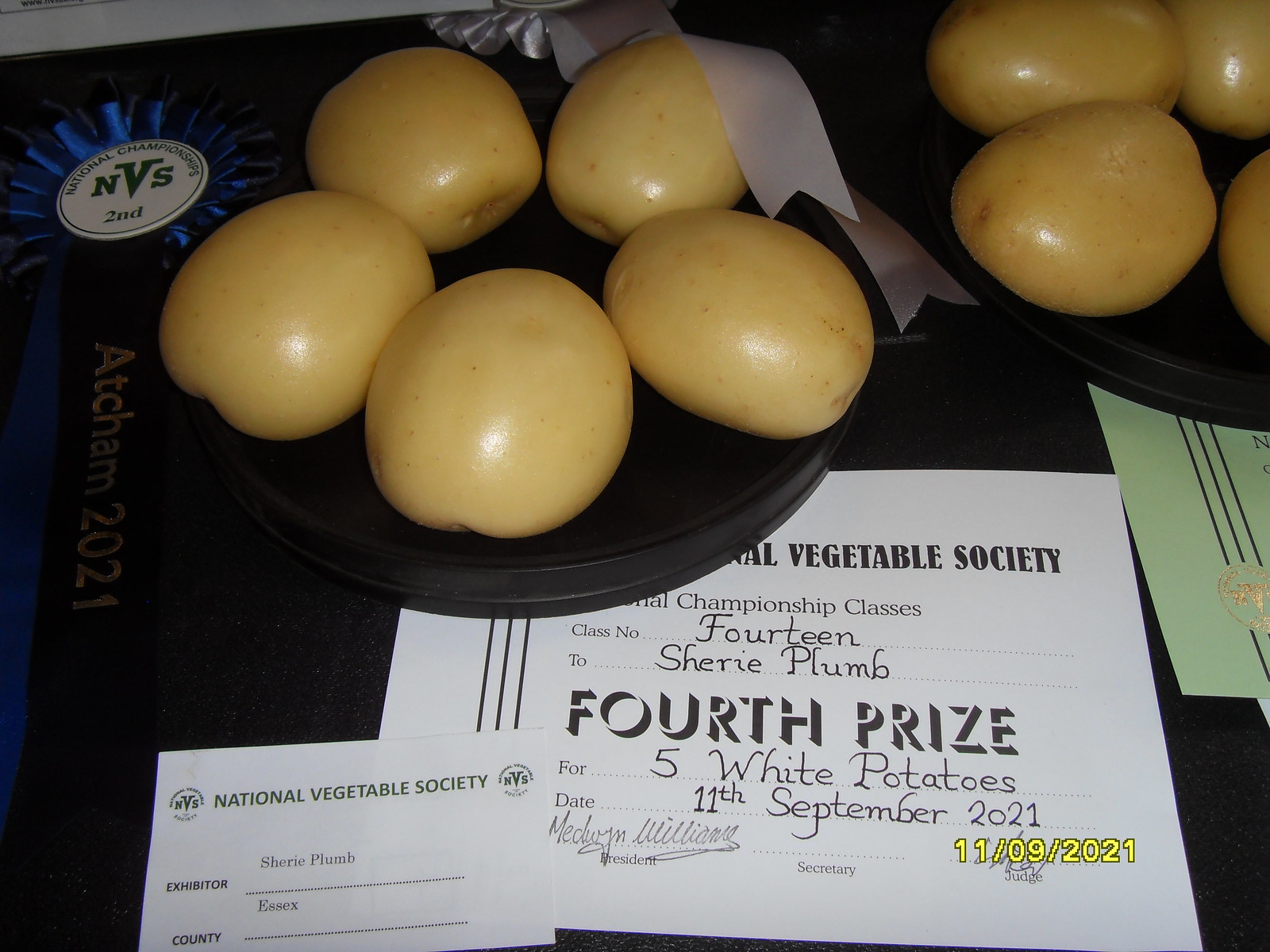The image is a detailed color photograph showcasing agricultural prize exhibits, specifically focusing on meticulously arranged potatoes and related award documentation. Central to the image is a black circular tray displaying five very neat and clean white potatoes. Positioned to the upper right is another similar tray, partially cropped, holding another set of potatoes. In the foreground to the left of the main tray, a blue second-place prize ribbon is visible, inscribed with "NVS National Championships, Second, ATCHM 2021" in gold text. Adjacent to the ribbon lies a small white card that reads "National Vegetable Society, Exhibitor Sherry Plum, County: Essex." Beneath the primary tray of potatoes, an official certificate is partially obscured, detailing the award: "National Vegetable Society, Championship Class, Class Number 14, Sherry Plum, Fourth Prize, Five White Potatoes, Date: 11 September 2021," signed by Medwin Williams, the president. In the bottom right corner of the photo, a digital timestamp marks the date "11-09-2021," consistent with the paperwork. This comprehensive snapshot captures the essence of a competitive vegetable exhibition, highlighting both the prestigious recognition received and the immaculate presentation of the potatoes.